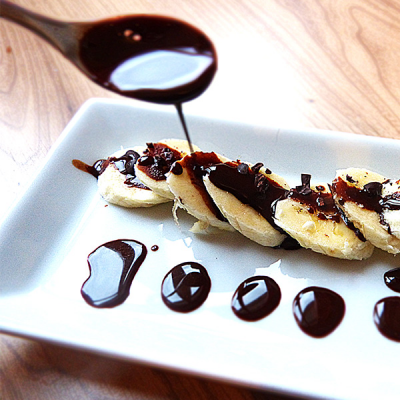The photograph showcases a carefully arranged dish of banana slices, meticulously laid out in a row, one on top of the other, on a rectangular porcelain plate. The plate is pristine white, placed on a light-colored wooden surface with prominent dark brown wood grain lines. A hand is in the process of drizzling a thick, dark chocolate liquid over the bananas, using a brown metal spoon. The chocolatier has artistically dropped small, circular dots of the same dark liquid adjacent to each banana slice on the plate. Additionally, the banana slices are adorned with shaved chocolate, adding texture and further emphasizing the rich chocolate theme. The overall image captures the elegance and precision of the dessert's presentation on the light wooden countertop.